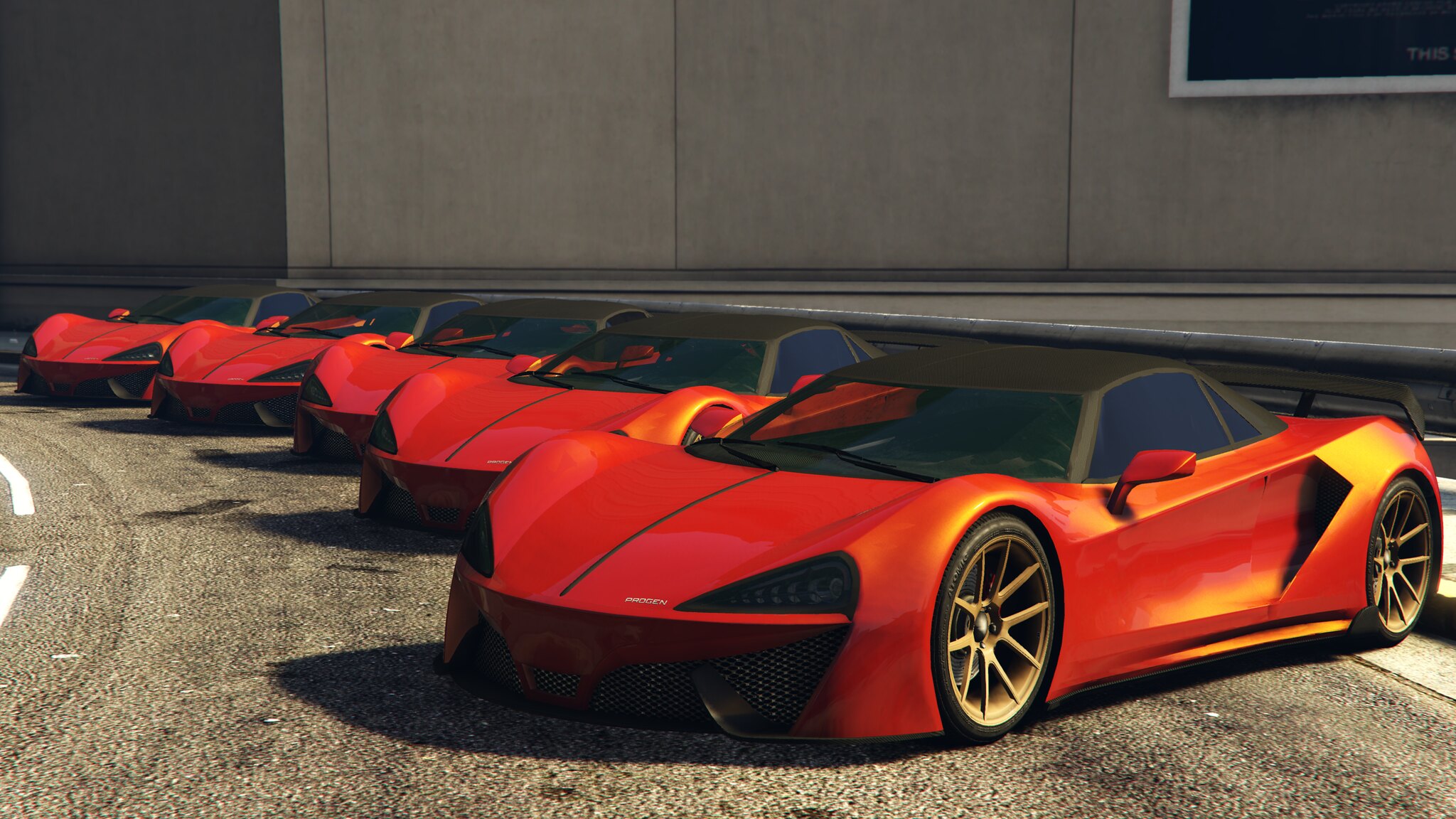In this digitally-styled outdoor image, five identical red sports cars, resembling Ferraris or Lamborghinis, are parked diagonally in a line along a curved asphalt road. The road features a broken white line in the middle and is closely bordered by a tall cement wall with a small white-framed window or sign in the top right corner, displaying the word "THIS" in white lettering. The cars, each equipped with a black convertible soft top, black spoiler, chrome wheels, and low-profile design, are positioned in such a way that only the front two cars are fully visible with their black spoilers. In the backdrop, a guardrail can be seen between the road and the building, adding to the detailed urban setting of the image.